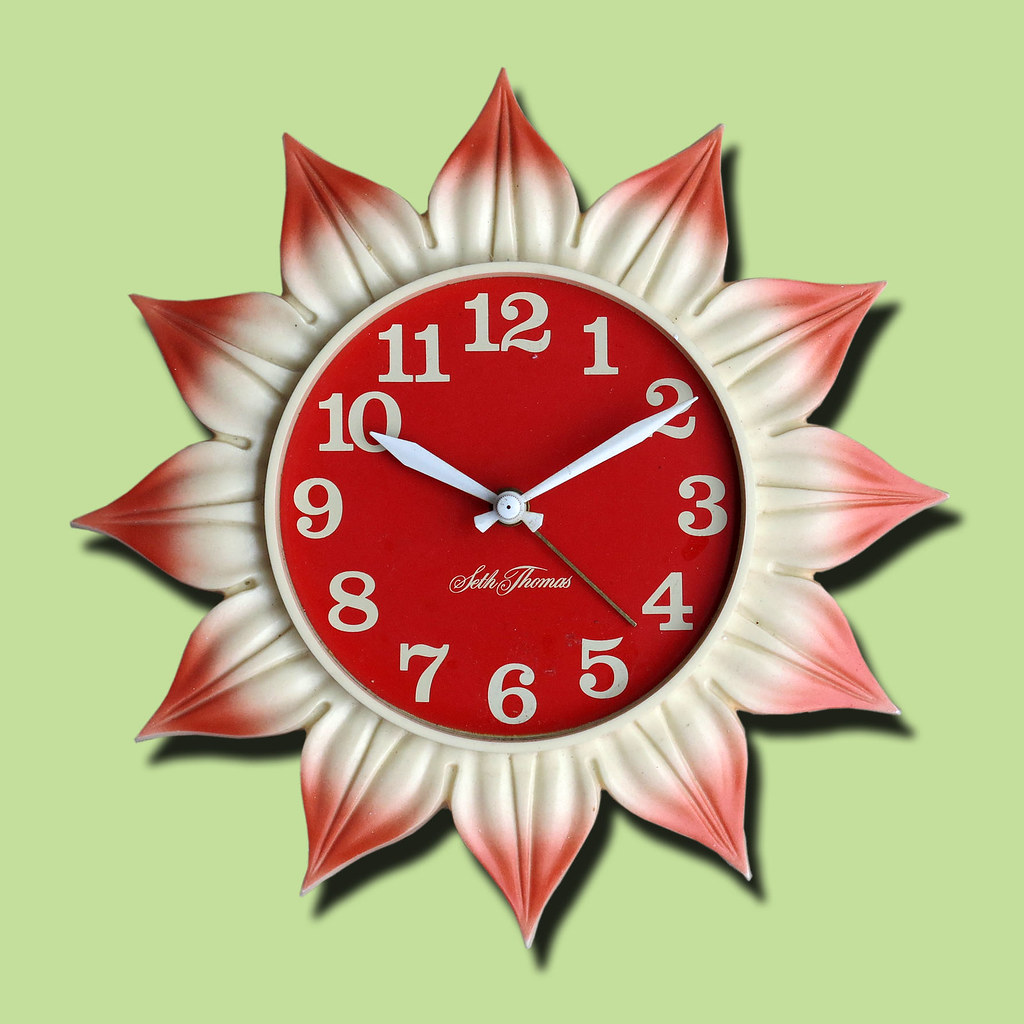This image features a centrally-placed, flower-shaped clock against a bright green background. The clock's unique design incorporates a white rim and a red face, with numbers one through twelve displayed in white. The hour and minute hands are also white, accompanied by a gray second hand. The words "Seth Thomas" are inscribed in cursive beneath the clock's hands. Surrounding the clock face, the flower's metallic petals are adorned with white centers transitioning into reddish tips through a fuzzy gradient. The clock's design casts a shadow, giving it a three-dimensional effect and making it appear as though it's slightly lifted off the background. The overall appearance suggests that the image might be digital, possibly sourced from an online game.